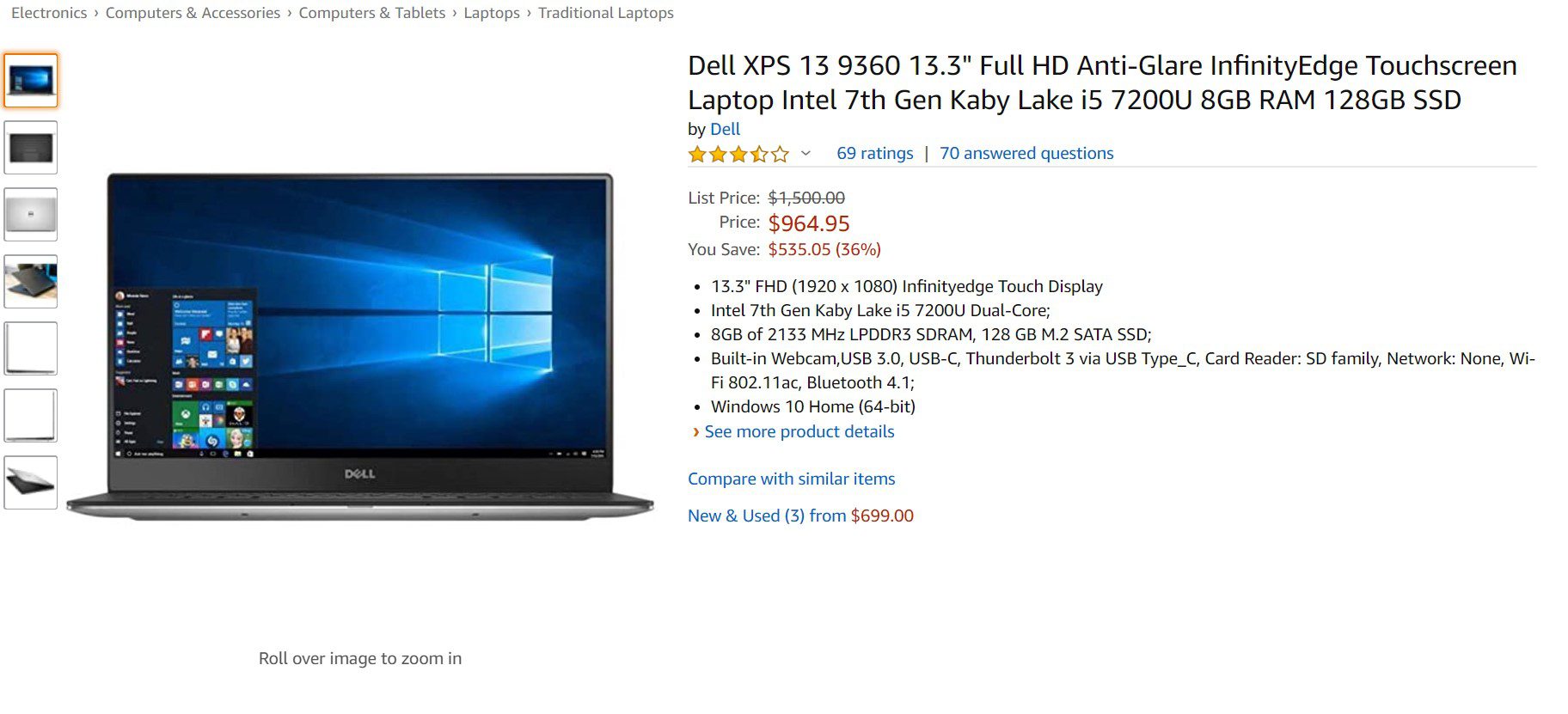This is a detailed screenshot of an Amazon listing for a Dell XPS 13 9360 laptop. The laptop features a 13.3-inch Full HD anti-glare InfinityEdge touchscreen. It is powered by a 7th Generation Intel Kaby Lake i5-7200U processor, endowed with 8GB of RAM and a 128GB SSD. The product image prominently displays the laptop with several smaller thumbnails showing various views, arranged on the left-hand side of the screen, totaling seven in number.

At the top, navigation breadcrumbs highlight the item's categorization progression: Electronics > Computer Accessories & Peripherals > Computers & Tablets > Laptops > Traditional Laptops. This listing has an average rating of 3.5 stars based on 69 customer reviews and features 70 answered questions.

Priced originally at $1,500, the laptop is currently available at a discount of 36%, reducing the cost to $964.05, resulting in a savings of $535.05. The main image highlights the laptop with its home screen active, including the visible taskbar. The rest of the image focuses on the laptop specifications and category navigation without other competing details.